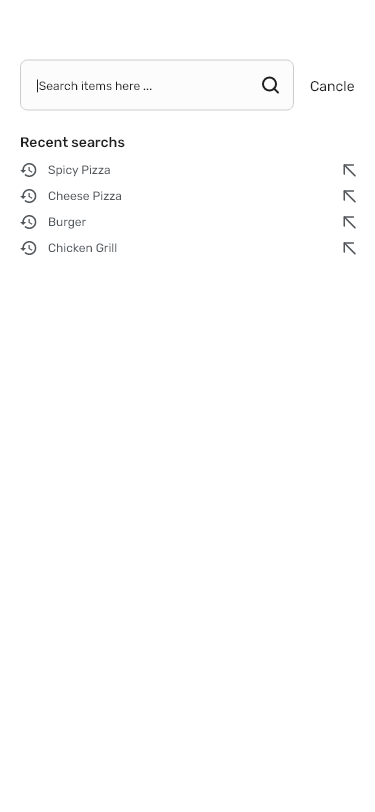The image features a minimalist search interface. At the top, there is a gray search bar with black placeholder text that reads "search items here..." To the right of the search bar is a magnifying glass icon representing the search function, followed by a misspelled "cancel" button labeled as "C-A-N-C-L-E."

Beneath the search bar, the heading "recent searches" appears, also misspelled as "recent searchs." Listed under this heading are four recent search terms: "spicy pizza," "cheese pizza," "burger," and "chicken grill." Each of these terms is accompanied by a gray clock icon on the left and a diagonal upward-pointing arrow on the right. The entire interface is set against a clean white background, giving it a simple and uncluttered appearance.